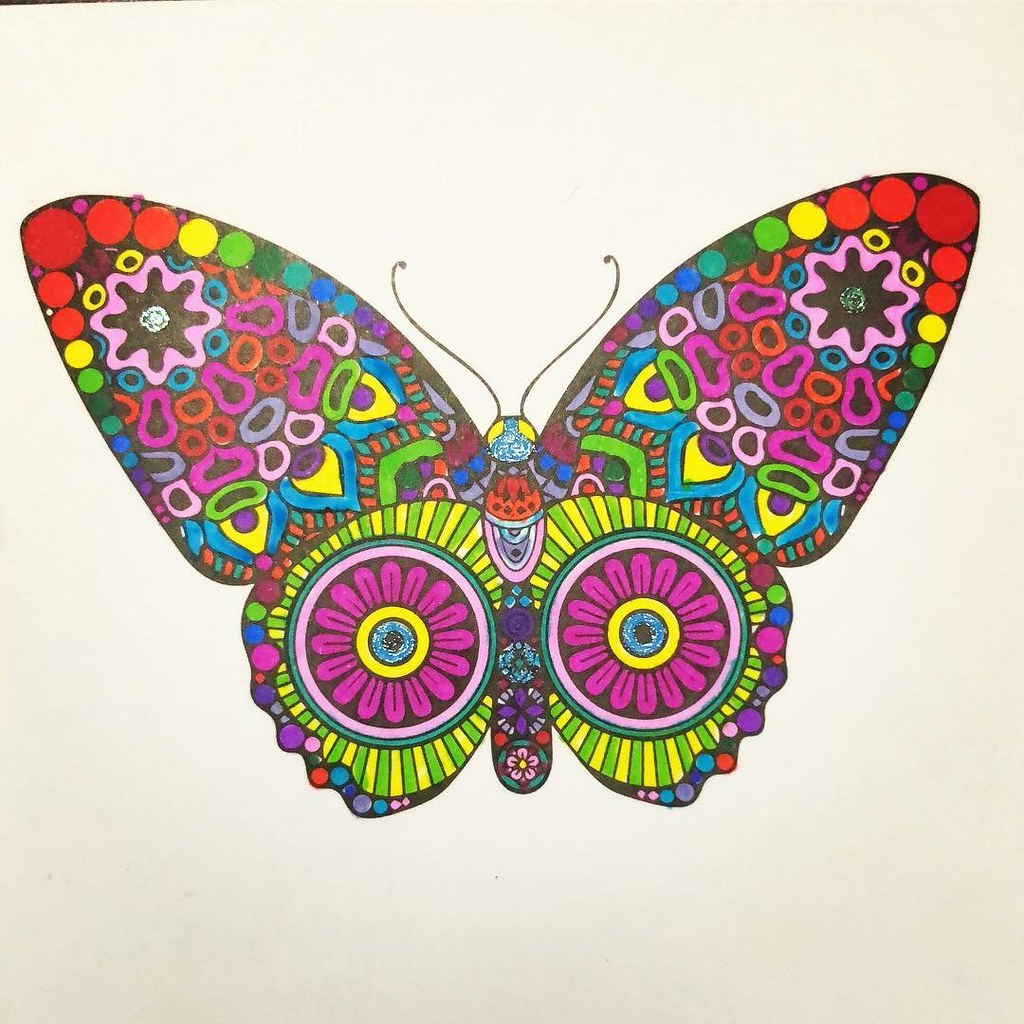This is a detailed and vibrant drawing of a large butterfly, occupying approximately 75% of the center of an off-white page. The butterfly is intricately outlined in black, featuring a mesmerizing array of bright and contrasting colors. The upper wings are adorned with a series of colorful circles—red, yellow, green, turquoise, and blue—forming a border around the edges. Inside these wings, there are distinct areas: a pink section with a black center, extended with white and circled by blue, displaying more blue circles interspersed with various shapes in pink, red, orange, blue, and yellow. Toward the base of the wings, a bright yellow merges with purple, framed by blue.

The body of the butterfly is equally detailed. It has two long black antennas protruding from a round yellow head with a blue center. The upper body transitions through red with black dots, and a pink area blending into blue and purple hues. The lower body or 'tail' is a striking purple, festooned with multi-colored circles. Extending from the body are yellow and green box-like patterns, each outlined in black.

At the heart of the composition is a pink flower, meticulously bordered by a pink line followed by a turquoise border. Inside these borders, yellow and blue are highlighted, all surrounded by tiny dots in vibrant colors like purple, red, pink, and yellow. This harmonious blend of intricate detailing and vivid color creates a dynamic and visually captivating artwork.